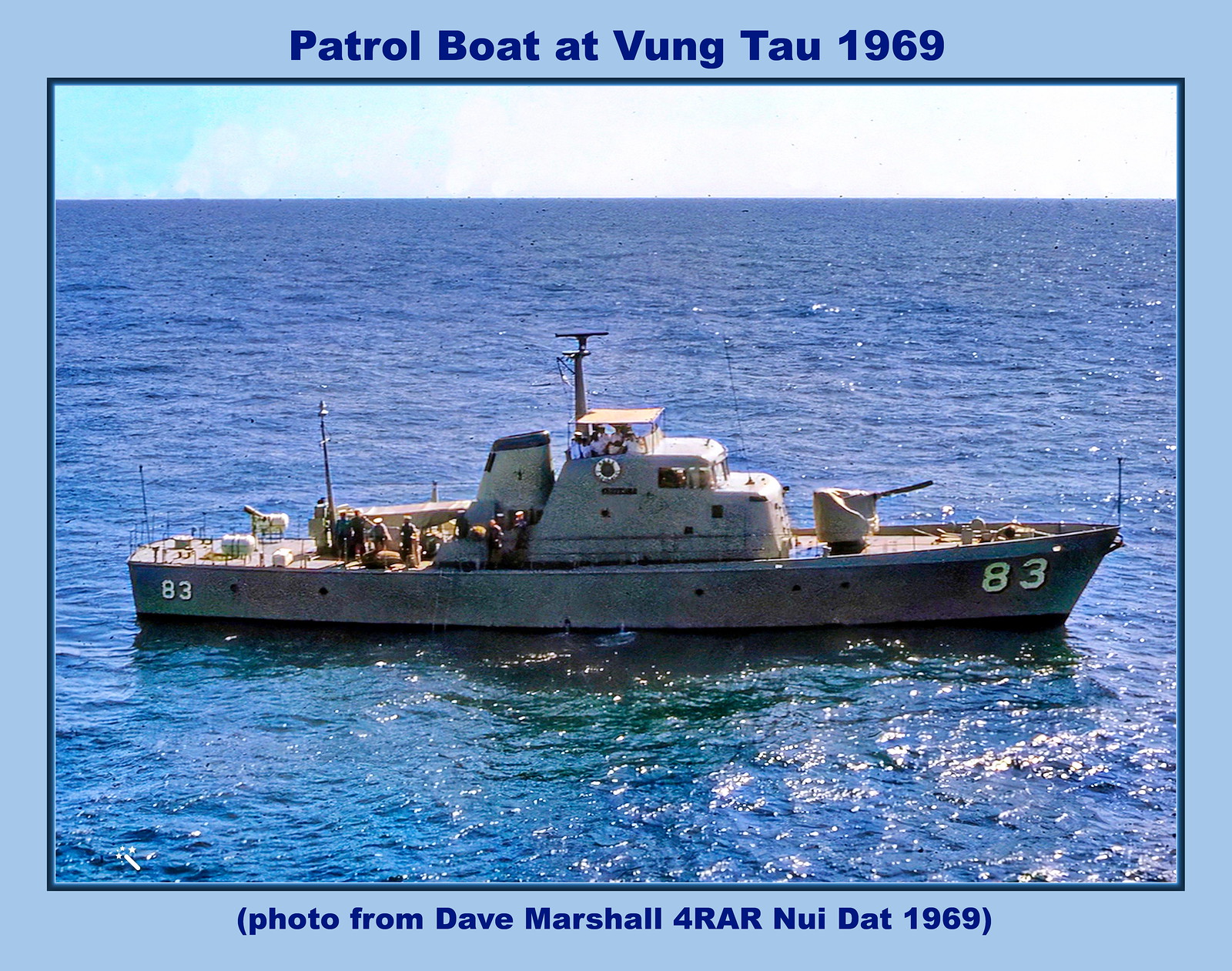The photograph captures a historical image of a military gunboat, identified by the number 83 prominently displayed on both the front and back of the white vessel. The boat is situated in the vast, bright blue ocean, under a similarly brilliant sky with scattered clouds, emphasizing the openness of the setting. It features a machine gun turret at the bow and equipment that appears to be radar or sonar above the deck where the captain's area is located. The scene suggests it is from the Vietnam era, specifically from 1969 at Vung Tau.

The picture is framed by a light blue border, with dark blue text at the top that reads "Patrol Boat at Vung Tau 1969." In matching dark blue text at the bottom of the border, it credits the photograph to Dave Marshall for RAR Nui Dat, 1969. The overall brightness of the image and the meticulous details suggest it might be intended for use in a book or on a website documenting historical military assets or events.